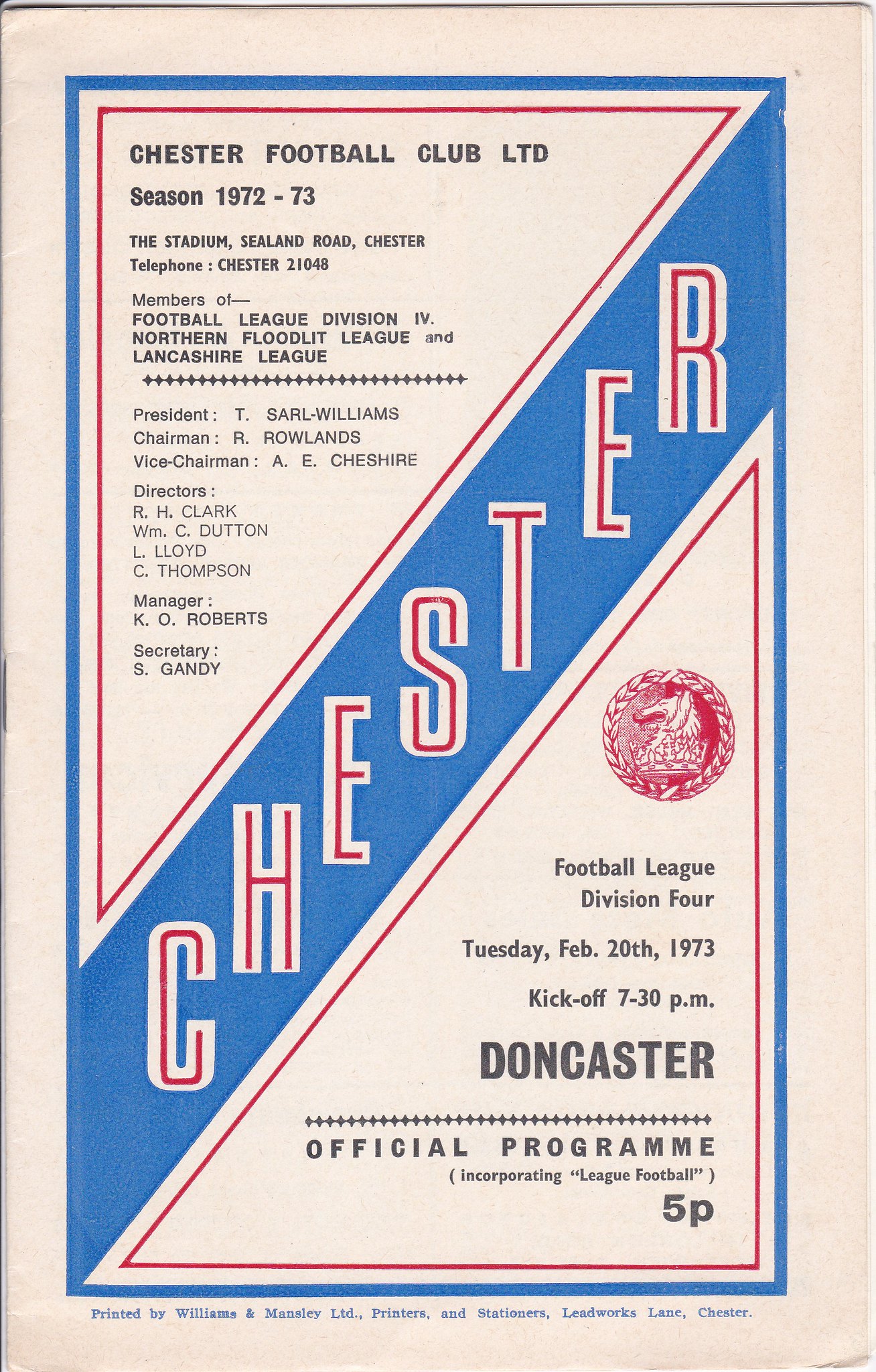The image showcases a vintage Chester Football Club LTD program from the 1972-73 season, meticulously preserved on cream-colored paper. It is elegantly framed by a royal blue border with intricate red detailing. Prominently displayed, the word "Chester" diagonally cuts across the page in bold red letters, bordered in blue, stretching from the bottom left to the top right. The text indicates that the club's home ground is Sealand Road, Chester, and includes a telephone number, Chester 21048. Chester Football Club is listed as a member of the Football League Division IV, the Northern Floodlit League, and the Lancashire League. The program details crucial information, such as key personnel: President T. Sarle Williams, Chairman R. Rollins, Vice Chairman A.E. Cheshire, Directors R.H. Clark, William C. Dutton, L. Lloyd, and C. Thompson, Manager K.L. Roberts, and Secretary S. Gandhi. 

A crest featuring a lion and a crown marks its official status. On the lower half, below the bold diagonal "Chester," more specifics are given: Football League Division IV match against Doncaster on Tuesday, February 20, 1973, with a kickoff at 7:30 PM. The program, priced at 5P, also credits its production to Williams & Mansley Limited Printers and Stationers, of Leadworks Lane, Chester. This well-centered vintage document captures the essence of the era, serving as a historical snapshot of Chester FC’s storied past.